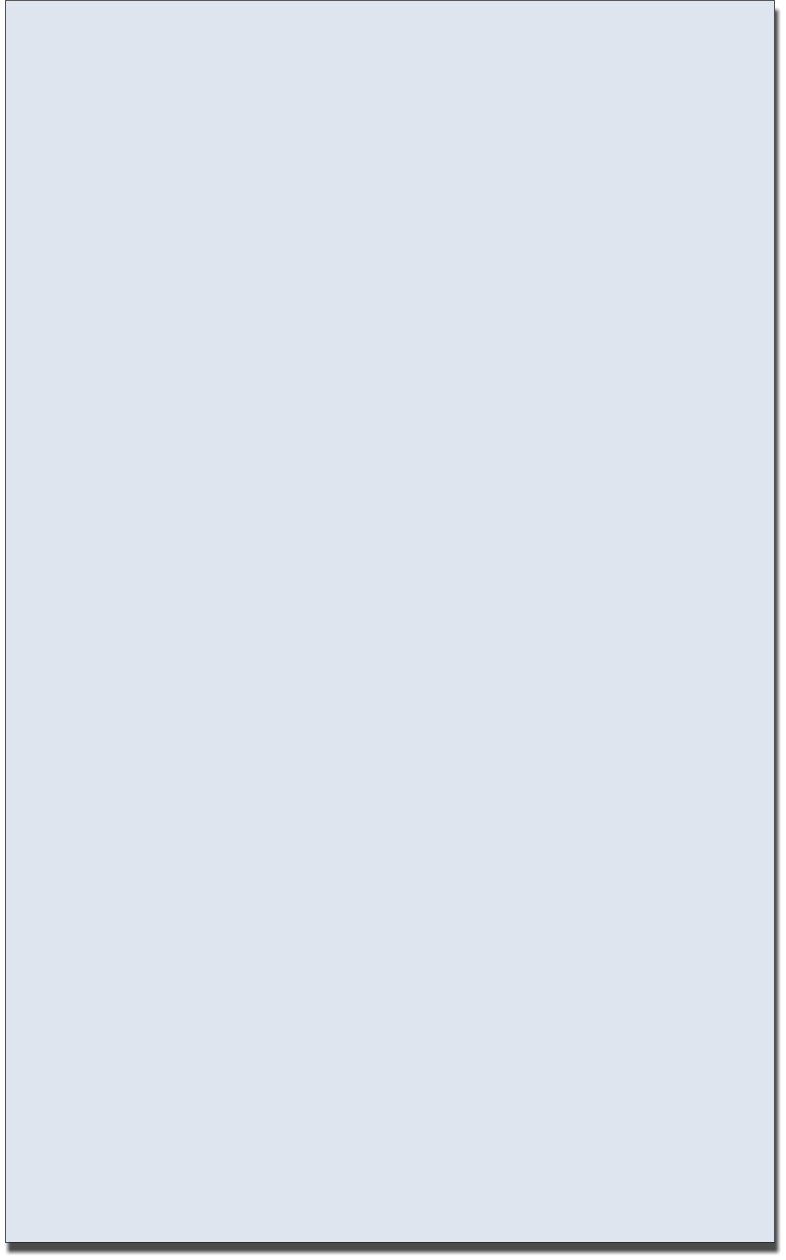The image portrays a seemingly blank page with a subtle bluish-gray hue. The page is bordered by a thin, grey line that runs across the top and down the left side. Towards the bottom left corner, the line transitions into a slightly thicker grey border that continues along the lower edge and all the way to the right side. The right border of the page appears marginally darker in comparison to the upper and left-side borders. The page is devoid of any text, people, websites, underlined elements, or links. When placed next to a white sheet, the page’s color distinctly appears as a muted greyish-blue.